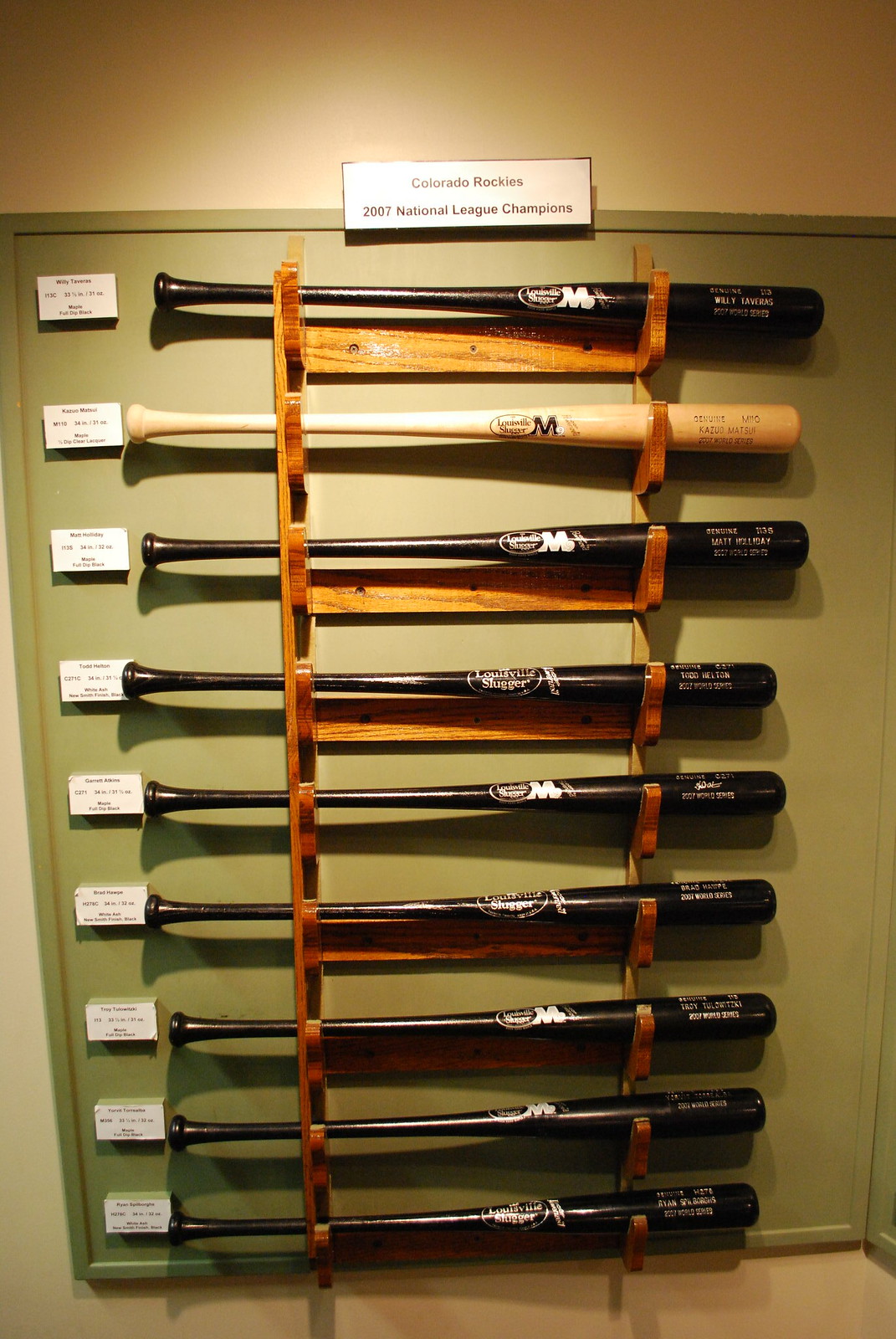This photograph features a display of nine baseball bats mounted on a green wall, backed by a brown wooden rack. The bats are arranged horizontally in a vertical line, with their handles pointed to the left and the barrels to the right. Eight of the bats are black adorned with a white letter 'M', while the second bat from the top is a lighter beige with a brown 'M'. Each bat has a small tag next to its handle, though the text on the tags is too small to read. At the top of the rack, a white plaque with black lettering reads "Colorado Rockies 2007 National League Champions," though the text appears blurry. The green wall has some molding accents, and a small section of the tan floor is visible at the bottom of the image. This detailed setup lends the appearance of a curated exhibit, possibly in a museum setting.